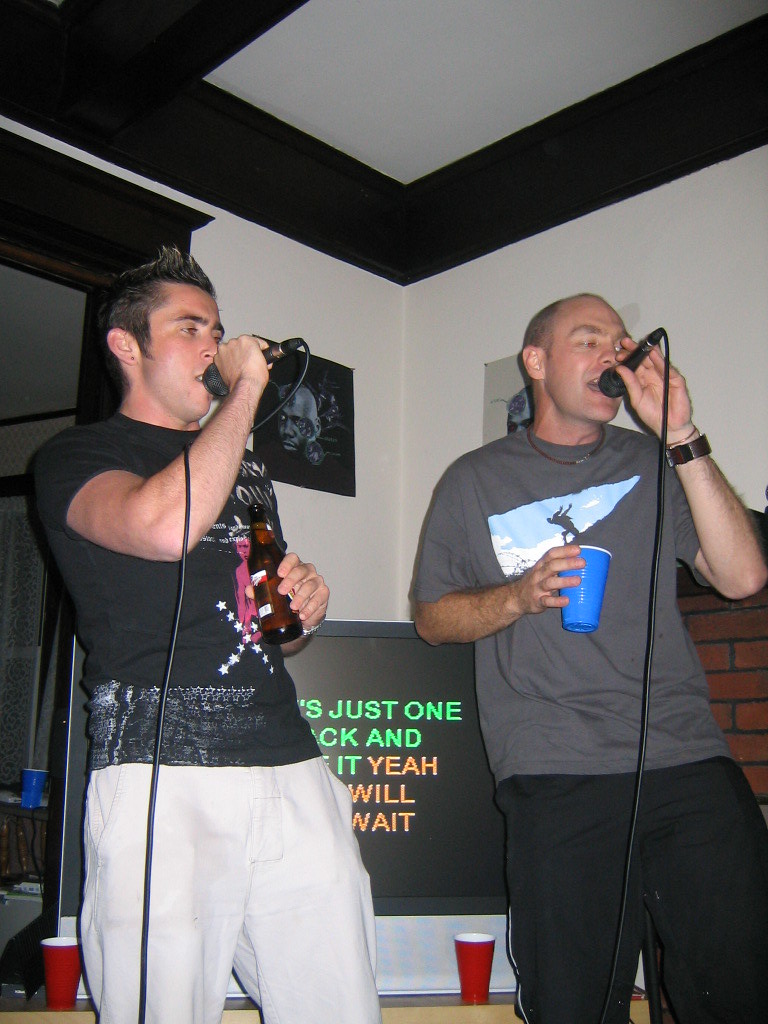This detailed photograph captures a lively scene of two men enthusiastically singing karaoke. They are positioned side-by-side, slightly to the right of the frame and facing forward, with microphones held to their mouths as they sing. Both are casually dressed in t-shirts and slacks, sporting short hair. The man on the left, who has slightly tanner skin and is wearing a black t-shirt, clutches a beer bottle in his left hand while singing into a microphone with his right. The man on the right, appearing slightly older and dressed in a gray t-shirt and black pants, holds a blue solo cup in his right hand and a microphone in his left. 

Behind them, a TV screen displays karaoke lyrics, with the phrases "just one..." and "...we'll wait" visible amidst a mix of sung words highlighted in green and upcoming lyrics in orange. The backdrop features white walls with wooden lining, a door leading to another room, and a section of brick wall or a fireplace partially visible. Red solo cups are scattered around, with at least two directly behind them, suggesting a casual party atmosphere. The room also includes pictures hanging on the wall and a mix of black and white ceiling portions. Both men appear fully engaged and are clearly enjoying themselves, contributing to the lively and spirited ambiance of the moment.